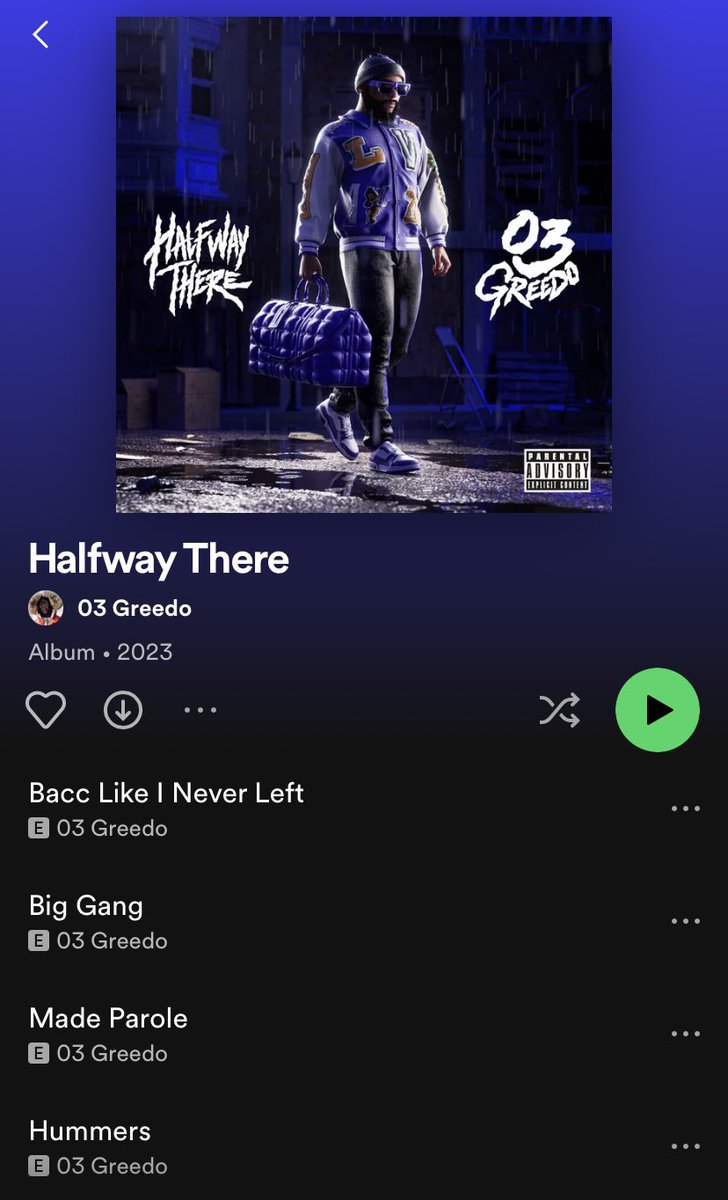This is a detailed screenshot of a Spotify playlist page. Dominating the top portion is an album cover centered within a gradient background that transitions from light blue at the top to a darker blue towards the bottom. Just below this gradient background, the interface shifts to a black theme that occupies the bottom half of the screenshot, where the song list is displayed.

In the center of this transitional area, there are several control buttons: a heart button on the left for liking the playlist, a download button next to it, followed by an ellipsis button. To the right, there is a shuffle button and a round green button featuring a play icon for playing the album.

The album cover appears again at the very top, and just below it, slightly offset to the left, the album title reads "Halfway There" by O3 Greta, released in 2023. A parental advisory warning is visible in the bottom right corner of the album thumbnail, indicating explicit content. Accordingly, each song listed in the playlist has an "E" denoting its explicit nature, positioned to the left of the song title.